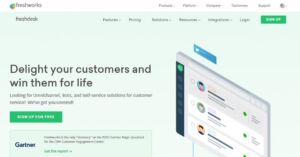The image features a predominantly green background with various textual elements. At the top part, set against a white section, there appears to be the phrase "Fresh Works," though it is somewhat blurry. On the far right of this white section, there are five black tabs, but the text within these tabs is too blurred to discern. 

In the upper left-hand side of the image, amidst the green background, there is a black text that reads "helped us." Adjacent to this area, on the right side, you can spot several black words, although they remain indistinct due to the blur. Below this section, there is a green rectangle containing white text, which could possibly say "Sign Up" or "Sign In," but this too is unclear.

On the left side of the image, in much larger and clearer black text, the words "Delight your customers and want them for life" are prominently displayed. Below this, the text shrinks again into an unreadable size. Further down the image, another green box is visible, possibly containing five words, but like much of the text in the image, they are too blurred to decipher.